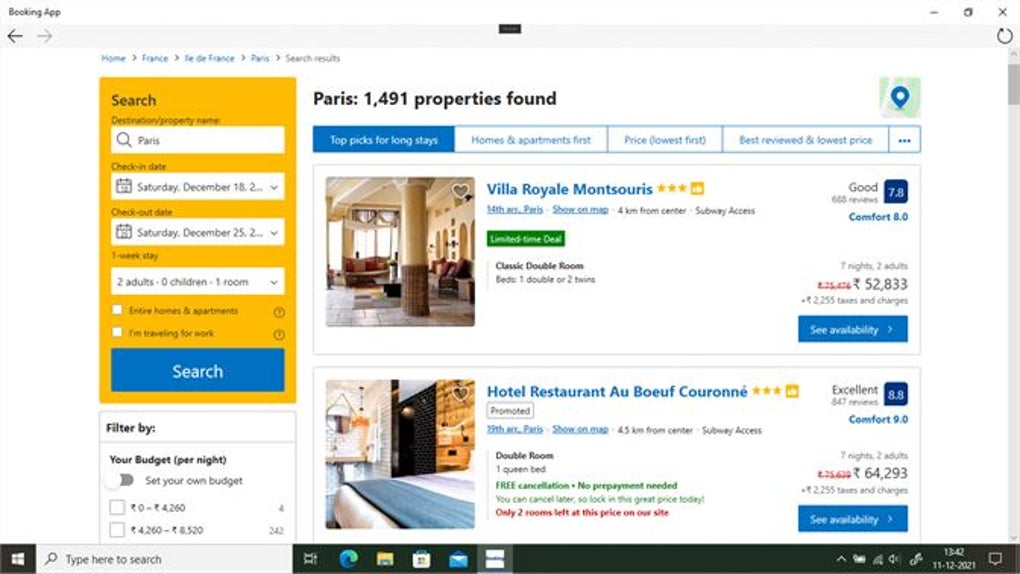This is a detailed screenshot of a travel booking website with a clean, white background. At the top center, in bold black letters, it reads "Paris: 1491 properties found." On the left side, there's a prominent yellow rectangle labeled "Search." Under the search section, the specified destination is "Paris," with a check-in date either on Saturday, December 15th or 18th (the number is unclear), and a check-out date on Saturday, December 25th. The search parameters include accommodations for two adults, zero children, and one room.

To the right of the search section, there are five filtering options displayed horizontally: 
1. Top picks for long stays (highlighted).
2. Homes and apartments first.
3. Price (lowest first).
4. Best reviewed and lowest price.
5. A small box with three dots indicating additional filters.

The listing section features two prominent options: 
1. "Villa Royale Montsouris," a three-star property marked as an ad.
2. "Hotel Restaurant Al Bof Corone" (name slightly unclear), another three-star property also marked as an ad.